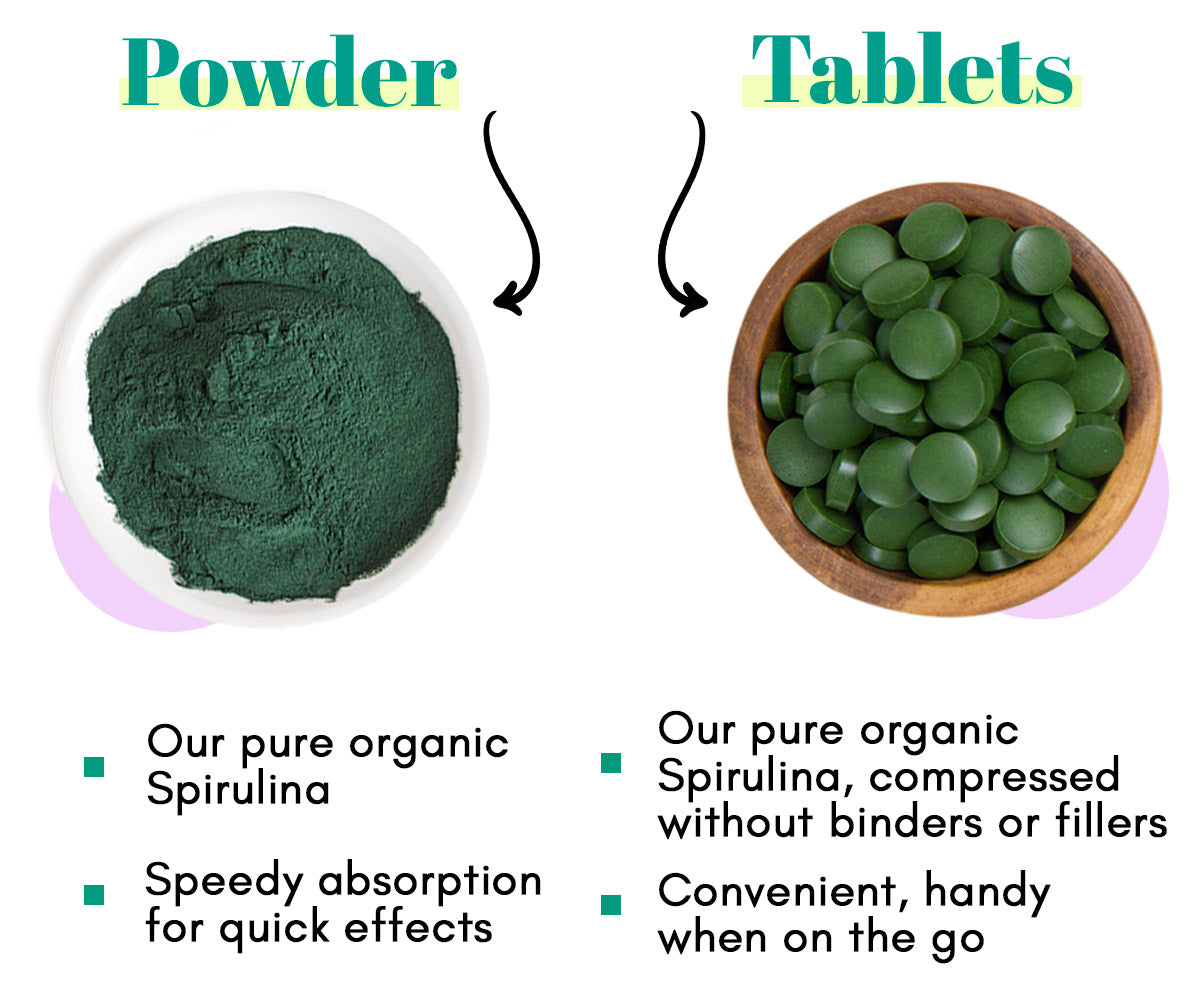The image is a comparison chart showcasing a product in two different forms: powder and tablets. On the left side, labeled "Powder" with a green label, there is a photograph of a white bowl containing green powder. A curvy black arrow points from the word "Powder" to the bowl. On the right side, under the green-labeled "Tablets," there is a wooden bowl filled with small, round, green tablets, with a similar arrow guiding the viewer from the label to the bowl. Above each bowl, there's a yellow line emphasizing the label. Underneath the "Powder" section, two bullet points highlight key benefits: "1. Our pure organic spirulina," and "2. Speedy absorption for quick effects." In the "Tablets" section, the bullet points state: "1. Compressed without binders or fillers," and "2. Convenient and handy when on the go." The entire chart uses photographs and black text on a white background for a clear presentation. Features like curving arrows and highlighted text further emphasize the distinctions between the two forms of the product.